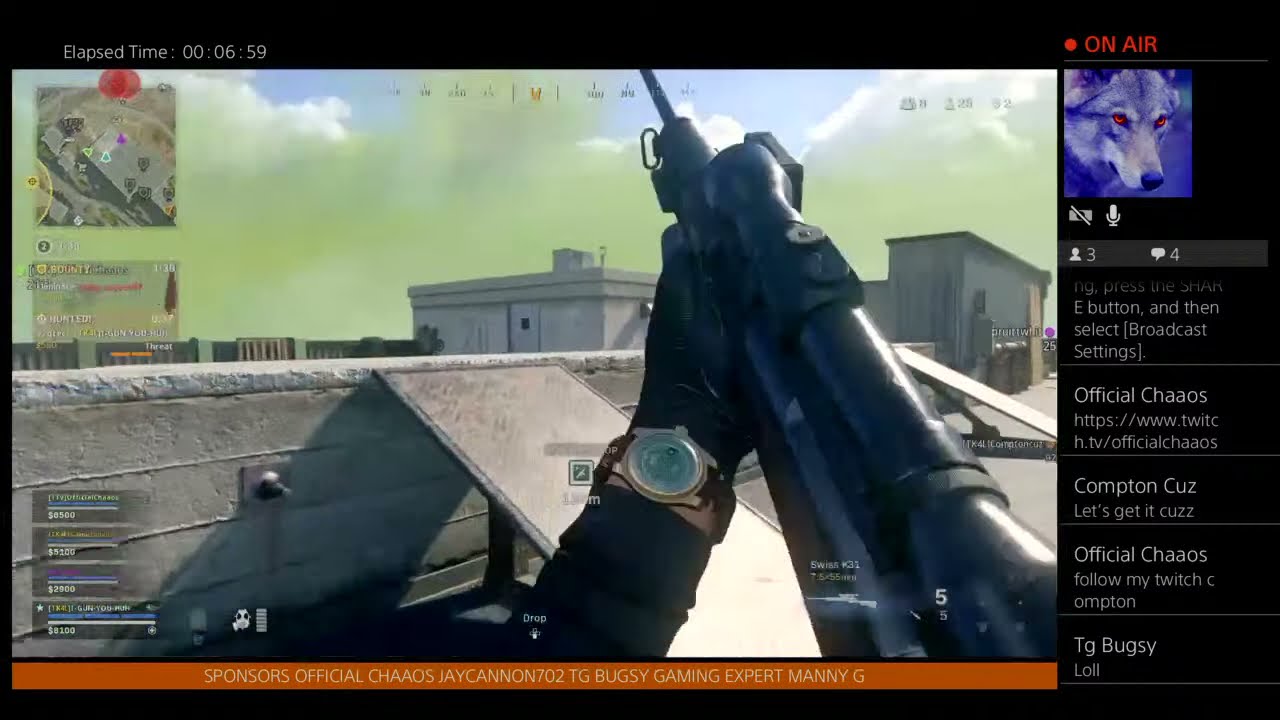In this detailed scene from a Call of Duty Warzone gameplay stream, we assume the perspective of the player holding a sniper rifle. The player’s left hand, adorned with a wristwatch and black glove, supports the gun, aimed towards the upper middle of the screen. We are positioned on the rooftop of the main prison building on the Rebirth Island map, with a wall to the left and the tops of other buildings visible in the distance. The sky is blue with streaks of greenish-white clouds. 

The streaming interface features black borders on the top right and bottom, enclosing the gameplay view. On the upper right of the screen, a red “On Air” indicator is accompanied by a wolf avatar with red eyes, showing three spectators and four comments below it. The upper left corner has a small map for navigation. A compass stretches across the top, and the bottom left corner displays another mini-map with squad stats.

An orange banner runs across the bottom displaying sponsor information: "Sponsors: Official Chaos, J Cannon 702, TG Bugsy, Gaming Expert Manny G." Furthermore, various overlay texts include “On Air”, “E button”, “Select Broadcast Settings”, “Official Chaos”, and “TJ Bugsy.” This setup indicates a professional stream powered by PlayStation, with an elapsed time stamp on the top left.